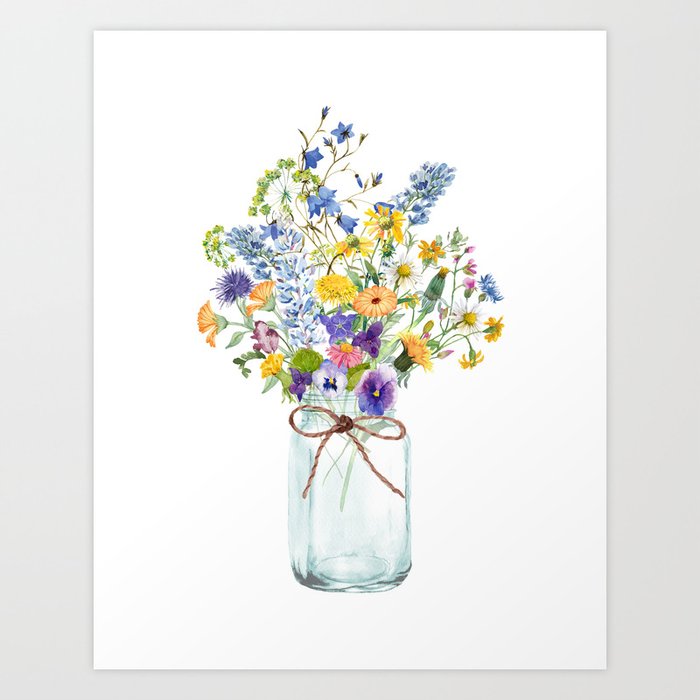This is a detailed watercolor painting depicting a vibrant floral arrangement in a glass mason jar, adorned with a brown jute ribbon tied in a bow around its neck. The diverse bouquet features an array of flowers in various colors including purple, pink, yellow, orange, and blue. Some of the flowers bear resemblance to marigolds and daisies, while others are less recognizable, adding to the eclectic beauty of the arrangement. The image is set against a stark white background, cropped from what seems to be a website, providing a clean and uncluttered frame that accentuates the vivid colors and intricate details of the flowers. There are no people or additional elements in the photograph, keeping the focus solely on the botanical subject.